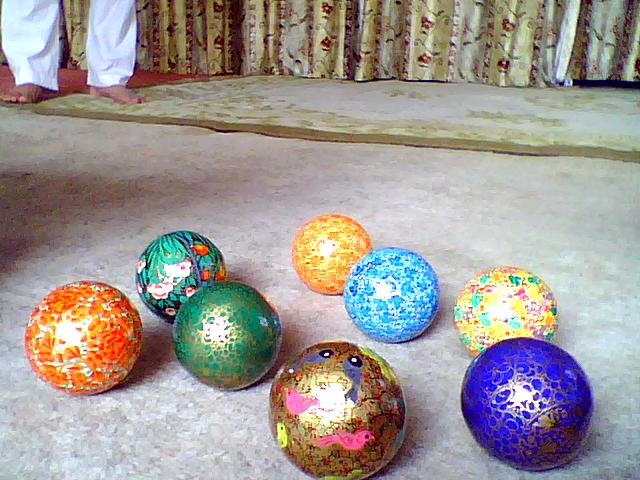The photograph showcases an assortment of eight intricately decorated ceramic balls arranged in the foreground on a beige carpet. The balls exhibit a wide range of colors and designs: an orange and yellow ball, a green, white, and orange ball, a green and gold ball, a gold ball adorned with pictures of birds and a fish, a yellow ball, a light and dark blue ball, a ball with green, red, yellow, and violet hues, and a dark blue and gold ball. Each ball is meticulously detailed, likely hand-painted, adding a sense of artistry to the scene. The setting suggests a living room, enhanced by the visible floor-to-ceiling floral-patterned curtains in a champagne gold color, and an additional rug in the background with an off-yellow hue and a brown border. A person, clad in white pants—possibly cotton or linen—and barefoot, stands partially visible to the upper left, while the photo, likely taken with a flash, captures reflections off the ceramic balls, illuminating the otherwise softly lit room.